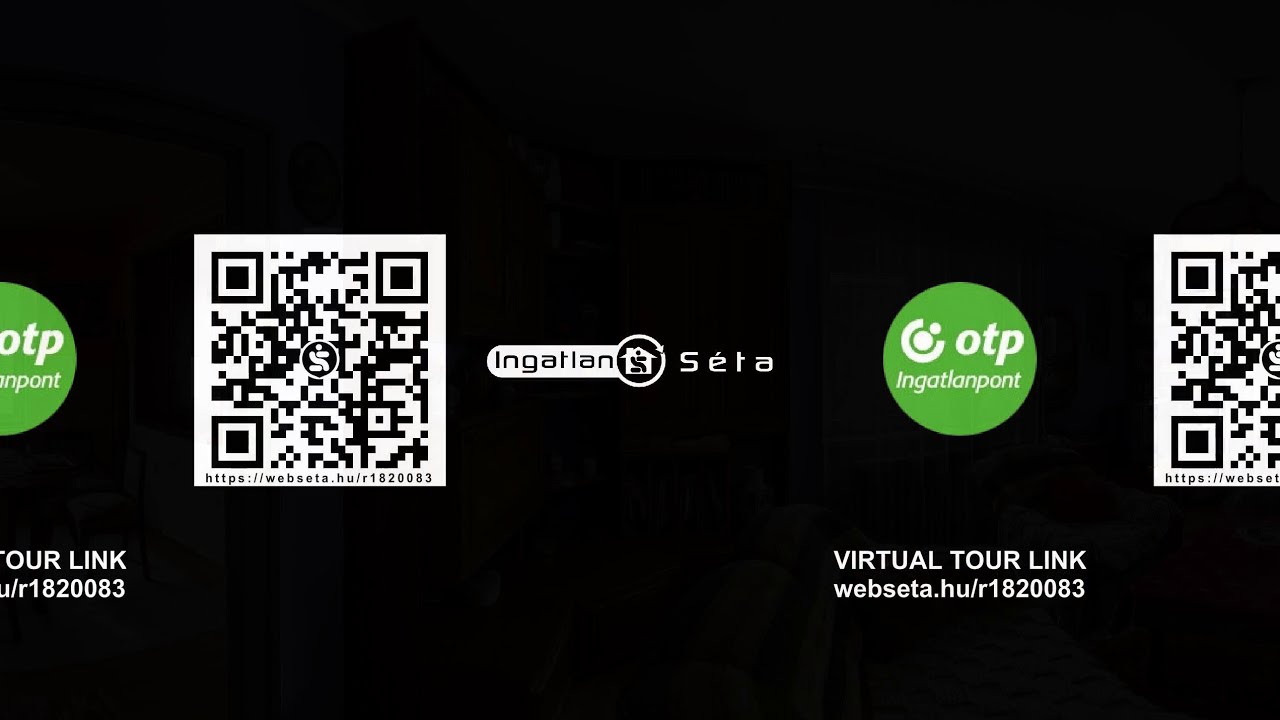The image features a digital advertisement set against a completely black background. Dominating the center is a large QR code with a logo in the middle, displaying a house icon and the text "Engation Seta" around it. Adjacent to this QR code is another logo, encased in a green circle with the inscription "OTP Engatlanpont." Below these elements, the text reads, "Virtual Tour Link: webseta.hu/R1820083." The overall color scheme is black, white, and green, and the elements are well-spaced, focusing attention on the QR codes and logos. The display appears to be from a website, likely Hungarian, as suggested by the URL and unfamiliar foreign text.